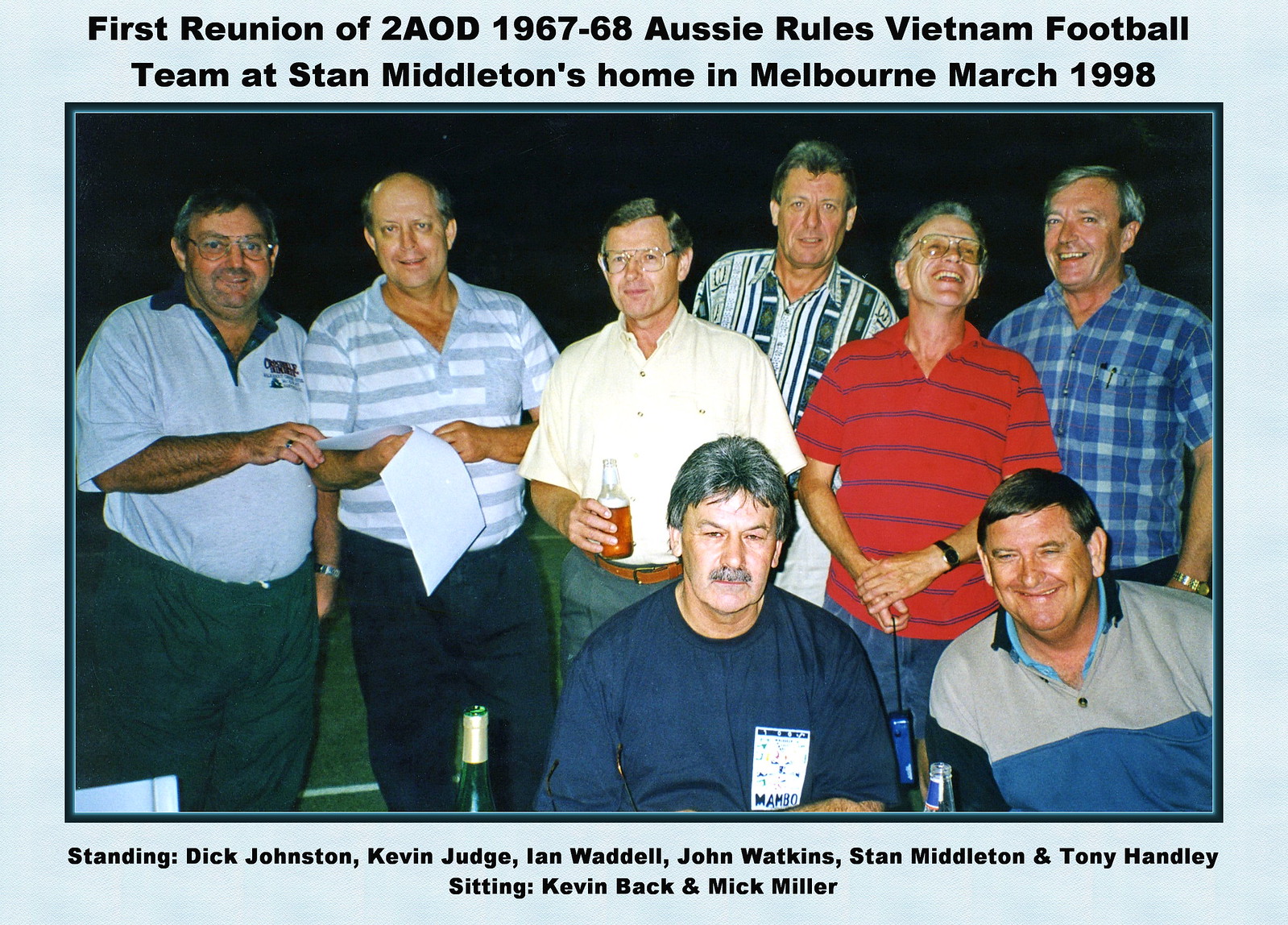In a photograph of the first reunion of the 2AOD 1967-1968 Aussie Rules Vietnam football team, taken at Stan Middleton's home in Melbourne in March 1998, eight men aged in their 40s or 50s are gathered, beaming at the camera. The image, set against a very light blue background, features text in black at the top reading, "First reunion of 2AOD 1967-1968 Aussie Rules Vietnam football team at Stan Middleton's home in Melbourne, March 1998." Below the photograph, another caption identifies the men in the order they are standing: Dick Johnson, Kevin Judge, Ian Waddell, John Watkins, Stan Middleton, and Tony Henley are standing, while Kevin Black and Mick Miller are seated. They appear to be enjoying themselves, some holding beers, reminiscing about old memories in a warm nighttime setting with a dark background and a touch of green below them.